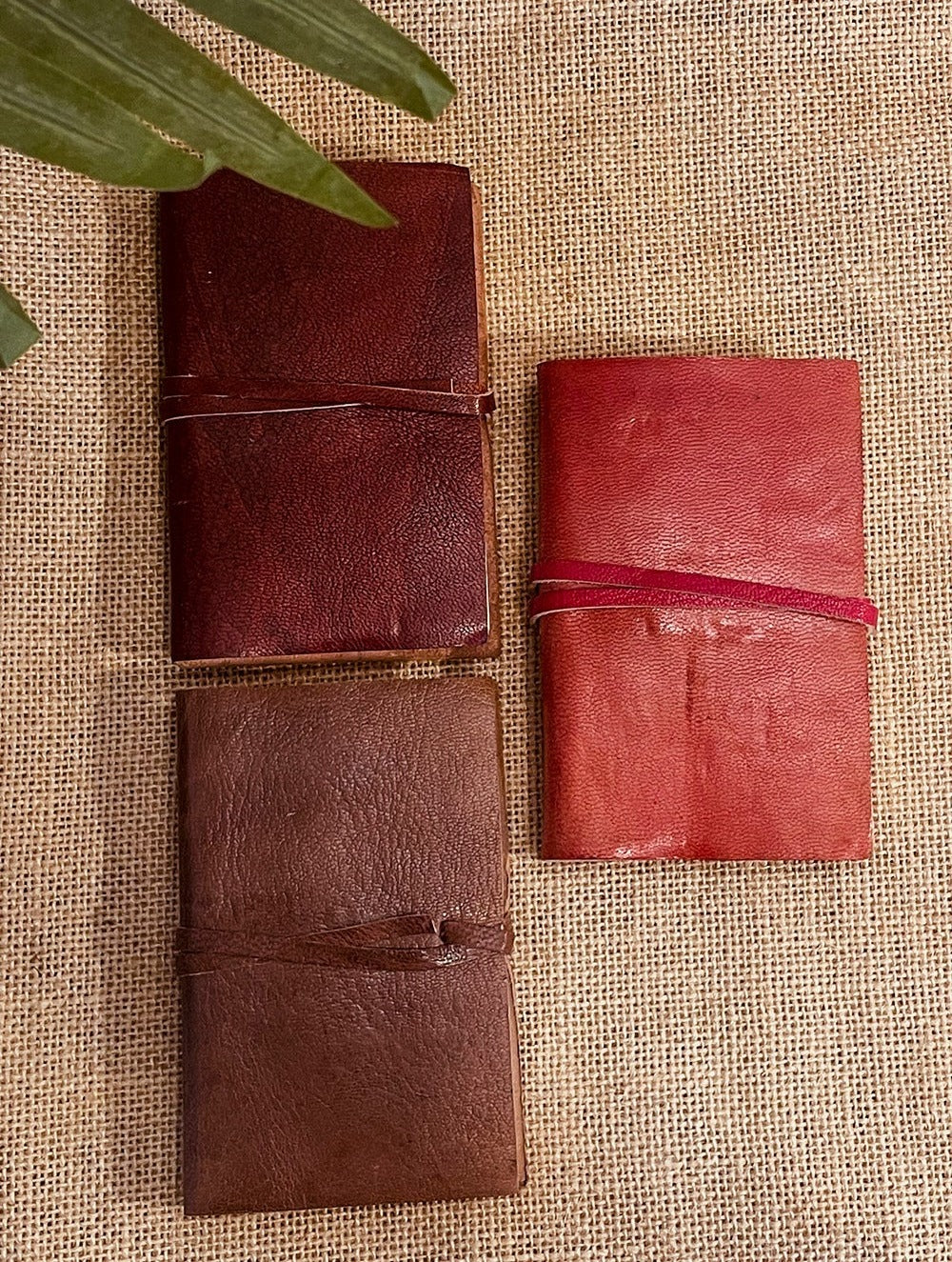Three leather-bound notebooks lie on a tan burlap canvas background, which has a rough texture similar to a sack. In the upper left corner, a few dark green leaves or grass blades peek into the frame. The notebooks, which appear handmade, are arranged with two on the left and one on the right. The leftmost column consists of a dark burgundy notebook, wrapped with a matching cord in the middle, resting above a medium brown notebook, also secured by a same-colored cord. To the right, a reddish notebook, tied with a leather strap a few shades darker than its cover, completes the trio. Though they resemble notebooks, they could also be mistaken for rectangular wallets due to their shape.